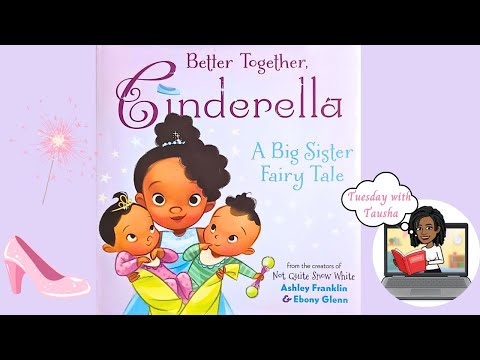The image appears to be a digital illustration, likely a promotional slide for a children's book. The top and bottom sections feature thick black borders, framing the main content. The background transitions from lavender to pink, then to light gray, and back to lavender. Prominently in the center is the partial cover of a children's book titled "Better Together Cinderella, A Big Sister Fairytale," showcasing a young African American girl in a blue dress, wearing a tiara, and holding two babies. One baby is in a pink onesie with a crown, and the other is in a green onesie holding a rattle. At the very bottom of the book cover, it credits the creators, Ashley Franklin and Ebony Glenn, noted for "Not Quite Snow White." The left side of the image includes a pink high heel shoe with a magic wand above it, while the bottom right corner depicts an open laptop with a cartoonish black woman emerging, holding a red book. A speech bubble from her reads "Tuesday with Tasha." This composite depiction emphasizes the storybook's theme and its enchanting, fairy tale aesthetic.